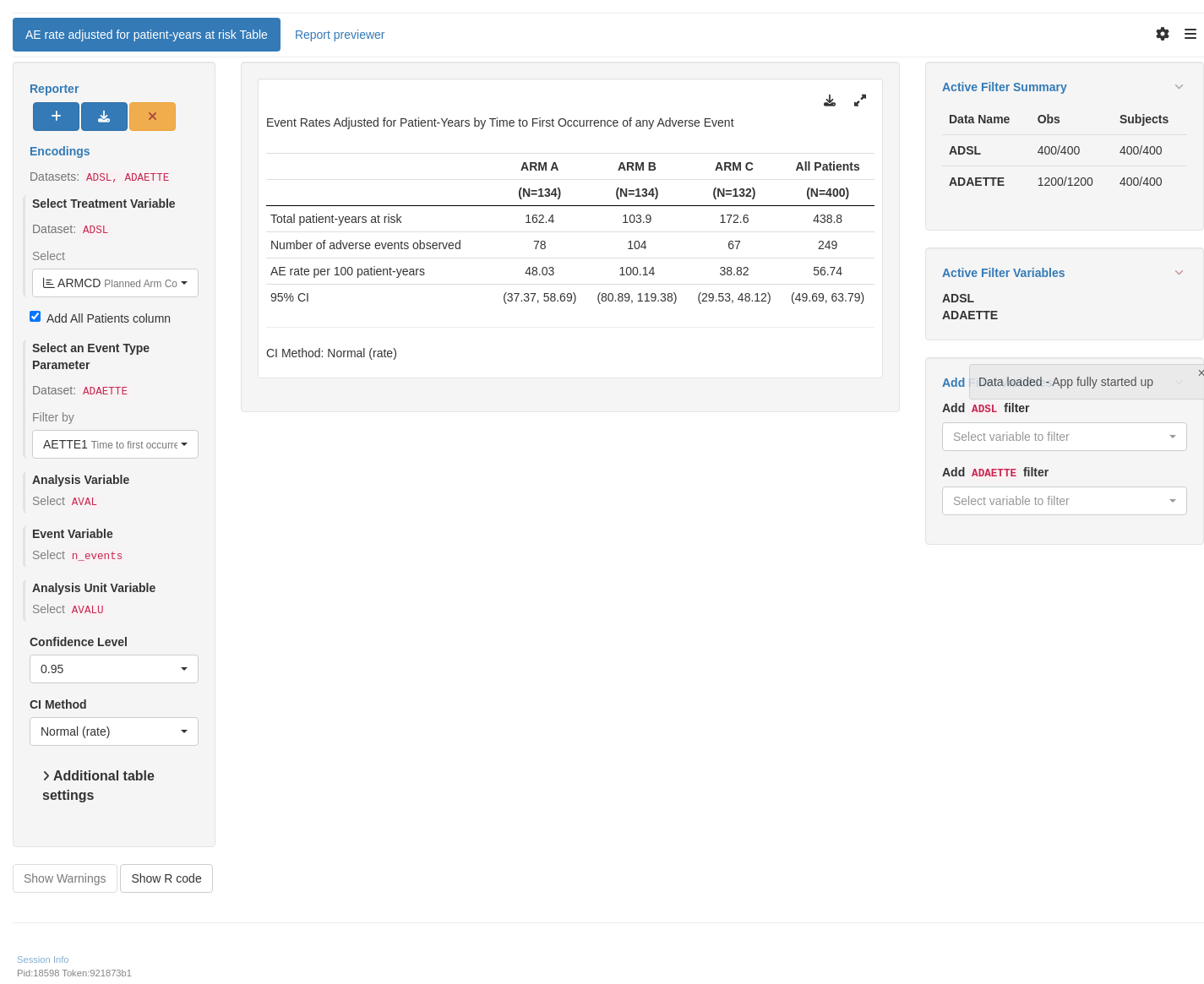The image features a predominantly white background populated with numerous small elements, each meticulously detailed. 

In the upper left corner, there’s a small blue rectangle with indecipherable white text inside. Next to this is another segment of text in blue, which stretches across to the right where it culminates into an emblem resembling a gear alongside three stacked horizontal lines.

Returning to the left, a long, light gray rectangle spans a portion of the image. It contains blue text, followed by a series of smaller, distinct rectangles: one blue with a plus sign, another blue rectangle with unrecognizable content, and a yellow rectangle adorned with a red X. Below these, a sequence of text appears in a complex array, beginning with blue words, transitioning through black and red text, and incorporating gray segments. 

Within this section lies a white rectangle bordered in gray, featuring black text and a square with a white checkmark. Adjacent to this are additional black words, followed by more black and intermittently red text. 

The lower portion displays multiple white rectangles containing numbers and text interspersed with tables and arrows pointing right. A light gray rectangle encapsulates another white rectangle filled with unreadable words and various symbols aligned to the top right, all appearing in black font. 

On the far right, several gray rectangles feature blue headers and black text. A slightly darker gray rectangle nearby contains text in black, although the words remain unclear. Below this, alternating sequences of words in black and red populate alongside white rectangles, creating a vivid, detailed tapestry of information amidst the minute content.